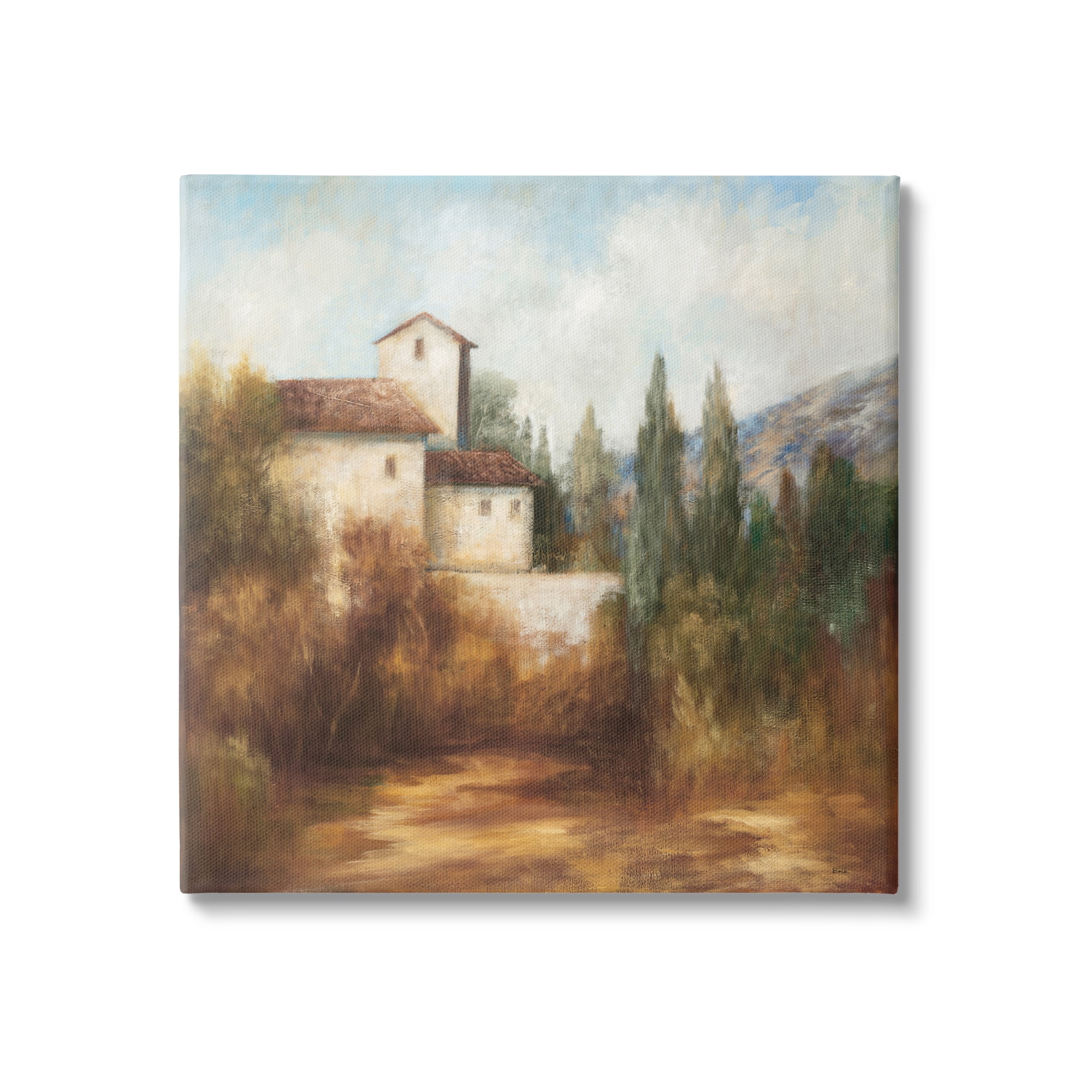This detailed painting, framed and displayed on a square canvas, portrays a serene countryside scene infused with a soft, faded palette and intricate oil painting techniques. The focal point is a stately, multi-storied white building, possibly a church or an elegant old house, characterized by its fragmented sections and terracotta-roofed extensions. The roofs, uniformly brown with slight accents, crown a structure adorned with a sparse number of windows, totaling four, creating a multitude of squares across its facade. The sky above is filled with soft white clouds against a blue backdrop, subtly transitioning into a majestic mountain range of oranges, blues, and whites towards the painting's right side. The landscape is peppered with tall trees, including evergreens, flanking a foreground of brown, dirt-laden ground interspersed with dead shrubs and older vegetation, enhancing the rustic charm of the scene. The overall Tuscan style imbues the image with a timeless, elegant tranquility.